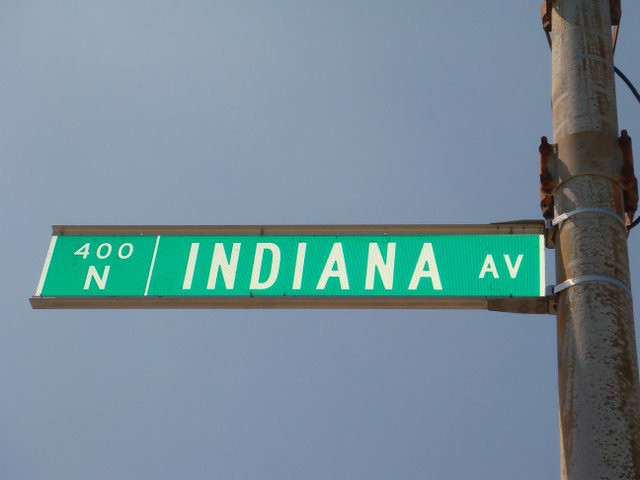This is a close-up photograph capturing a rectangular street sign in a landscape orientation. The sign prominently displays "400N Indiana AV" in bold white lettering, set against a vibrant green background. The top and bottom edges of the sign feature a gray border. To the right, a gray pole, adorned with two light gray plastic fastenings, secures the sign in place. The backdrop of the image reveals a sky tinged with dark bluish-gray hues, adding a dramatic contrast to the scene.